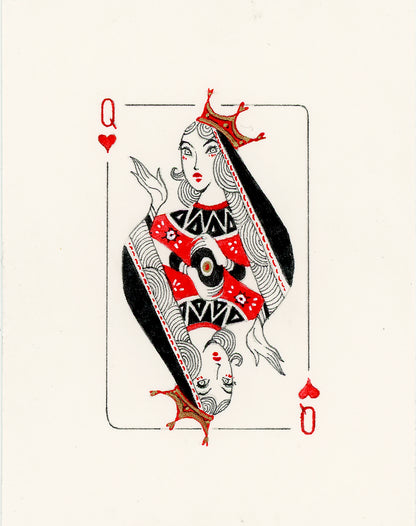The image depicts the Queen of Hearts playing card from a deck. The card’s background is an old, off-white color bordered by a thin black line. In the center, a mirrored illustration features the queen both upright and upside down. She has a white face, adorned with red lipstick and red accents under her eyes. Her attire includes a red dress with intricate white designs, and a black collar patterned with white triangles. Over her curly hair, the queen wears a red crown with gold details and a long black veil. Her hands hold a black, white, and red wheel at the center of the card. The corners of the card display a red 'Q' and a red heart, positioned at the top left and bottom right, respectively, with the top representing the card’s upright position and the bottom its inverted reflection. The overall presentation conveys a timeless, slightly worn appearance, characteristic of a well-used deck.